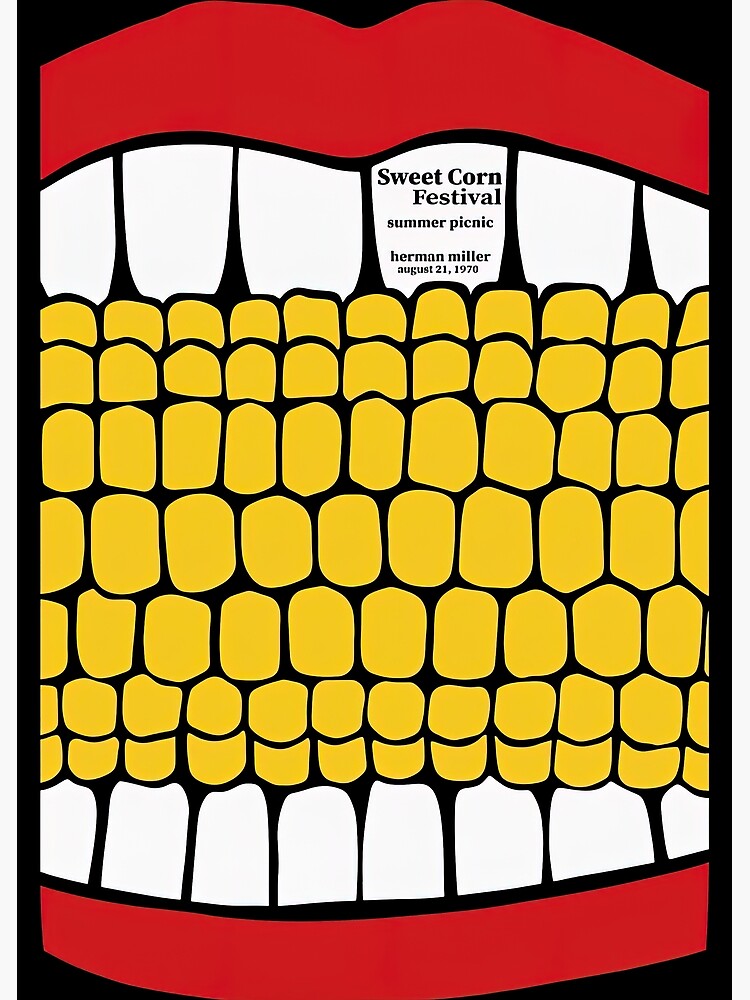The poster is a vibrant, stylized illustration promoting an upcoming event. Dominated by an image of a mouth in the act of biting down on an ear of corn, the piece features flat, bold colors without photorealistic shading. The large, ruby-red lips frame the top and bottom of the artwork, enclosing pure white teeth and a thick ear of yellow corn. The corn is meticulously detailed, with seven rows and eleven columns of kernels. The mouth appears to be eating the corn, and on the fourth tooth from the left, the event details are written in clear text: "Sweet Corn Festival, Summer Picnic, Herman Miller, August 21st, 1970." The entire image is outlined in a thick black border, enhancing the graphic and eye-catching quality of the design.